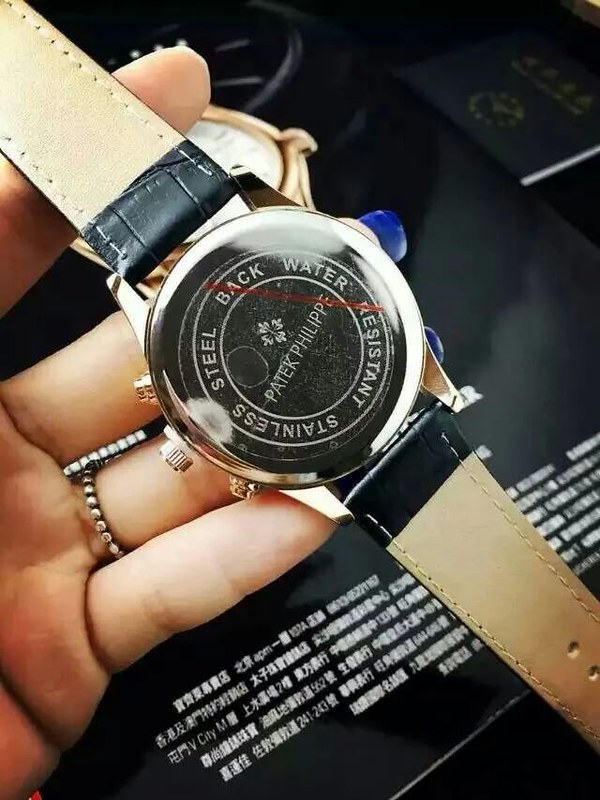In the image, a female hand is prominently featured, emerging from the left-hand side. The hand holds a watch, displaying the back side of the timepiece. The person wears a ring on their ring finger, and the tan leather watch band, adorned with some black markings near the watch face, is draped elegantly across her fingers. The back of the watch is black and inscribed with several pieces of text: around the perimeter, it reads “Backwater Resistant” and “Stainless Steel,” while the center is marked with the prestigious brand name “Patek Philippe.” The backdrop of the image is a black surface, possibly paper, which includes some white writing in Chinese characters, adding an element of cultural intrigue. The details of the Chinese text are not discernible.